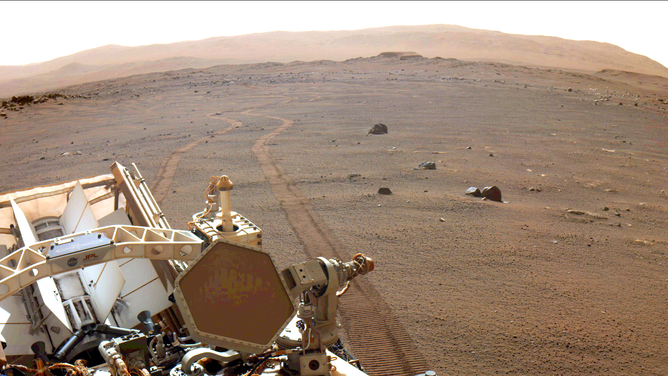The photograph captures a section of a Mars rover amidst the vast, flat, and desolate Martian landscape. The dominant colors in the scene are various shades of brown and red, characteristic of Mars' dusty surface, interspersed with sporadic large black rocks. The lower left of the image prominently features an intricate portion of the rover's machinery. This machinery includes white and metallic components, some of which appear to be part of a solar panel, along with numerous wires and mechanical parts. A distinctive red, octagon-shaped panel is noticeable on the machinery. The Martian terrain in the background reveals faint mountain ranges under a washed-out sky, and the ground bears the clear, meandering tracks left by the rover, emphasizing its journey across this barren, plantless desert.